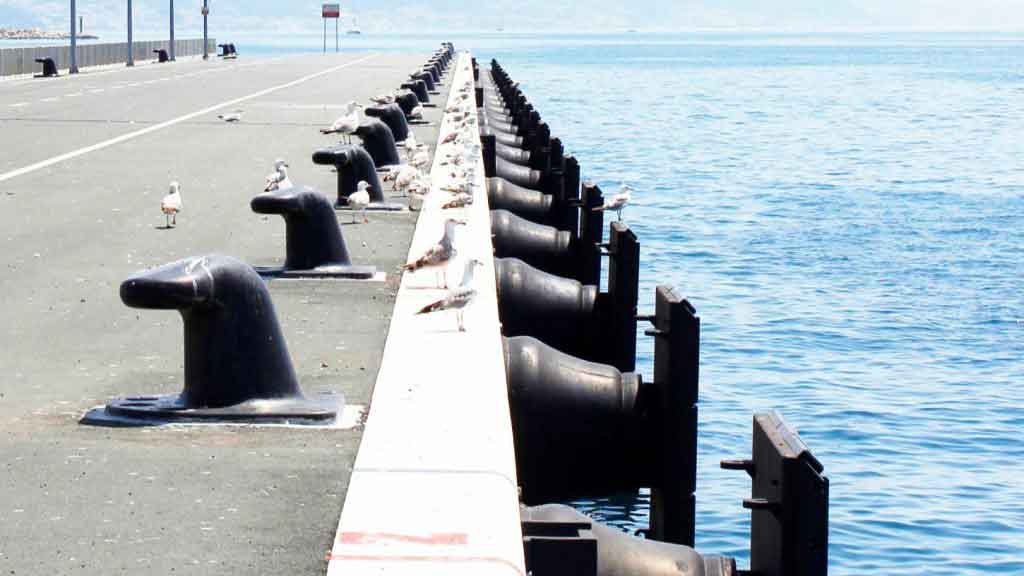The image showcases a pier extending into a vast, calm body of blue water, possibly an ocean. The pier is populated by numerous seagulls, predominantly aligned along the right-hand edge, which features a distinct white-painted strip. This strip is part of the concrete cement structure of the pier. Along the length of the pier, there are several robust, black, bell-shaped bumpers bolted down, designed to cushion large vessels such as shipping or cruise ships. These bumpers have vertical rubber-coated ends providing additional protection. Additionally, there are rows of short, large metal tie-down structures shaped like submarine tails, used for securing docked ships. The left side of the pier appears to be adjacent to a paved road or street, with more seagulls and similar structures along its edge. At the distant end of the pier, a red sign is visible, though too far to discern details. The scene is bathed in daylight with minimal wave activity, adding to the tranquil ambiance. In the blurred background, one can faintly make out land or another part of the dock, completing this nautical setting.